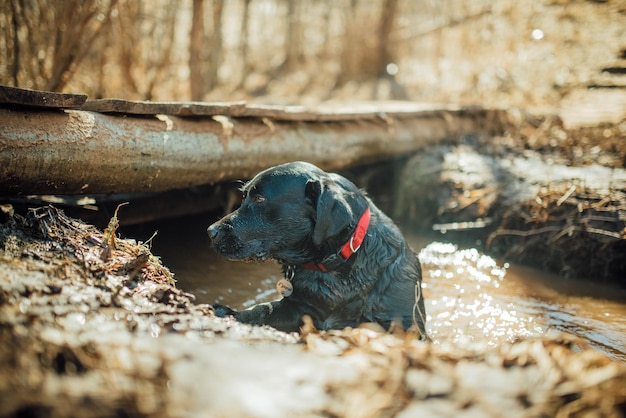This horizontal rectangular photographic image captures a black dog, potentially a black lab, positioned near a creek bank in an outdoor, wooded setting during daylight. The dog, which is wearing a red collar with a silver buckle and an unreadable silver tag, is in profile, gazing to the left. The foreground showcases a mix of wet brown soil and water, suggesting the dog might be partially in the stream. Directly behind the dog, a rustic log bridge comprised of logs and planks spans the creek. The background features an out-of-focus view of tree trunks, adding to the natural ambiance. Sunlight hits the water, illuminating parts of the image and lending a generally brown hue to the scene, contrasting with the dog's darker fur.